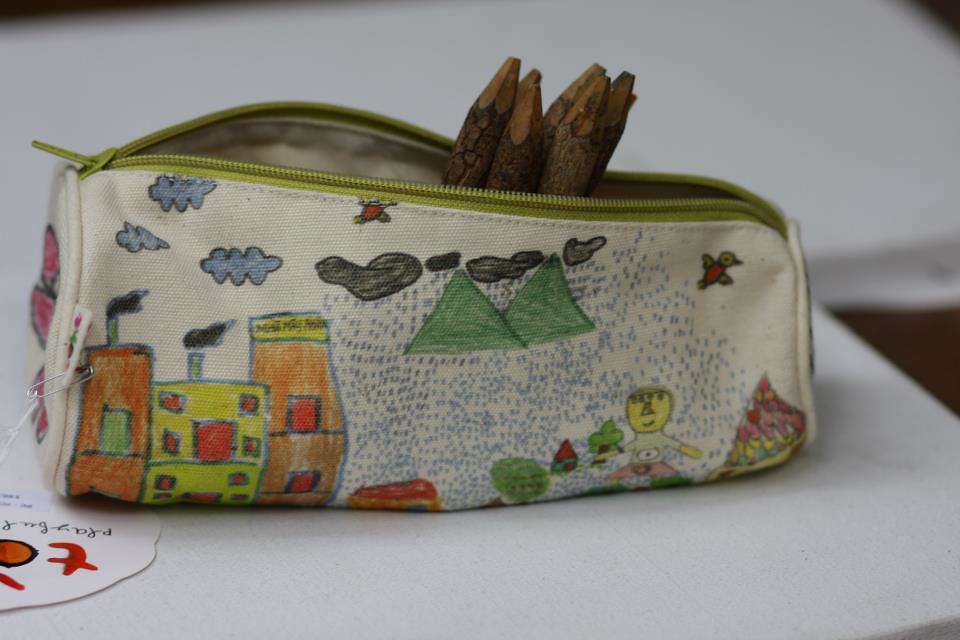The image showcases a small, cream-colored canvas pencil case with a green zipper, lying on a smooth white surface, possibly a table or countertop. The pencil case, which is oriented horizontally, is partially unzipped, revealing around five twig-like pencils with bark still on them, resembling whittled branches rather than conventional pencils.

The canvas material of the pencil case is adorned with childlike drawings, possibly done with colored fabric markers. These illustrations feature three multi-story buildings on the left, two with chimneys emitting smoke. The buildings are primarily orange and green with variously colored windows. Above the buildings float black-outlined blue clouds amidst green triangular shapes reminiscent of mountains, which appear to be floating due to the light-colored canvas background. The clouds exhibit falling blue raindrops scattered across the bag.

Additionally, two small, colorful birds—red with yellow and perhaps greenish wings—are depicted flying in the sky. Towards the bottom of the bag, a small yellow figure with a triangle nose, a little fringe of hair, and a smile is visible, seemingly dressed in pink shorts. A tag attached to the pencil case reads "playful" and possibly more wording starting with "T-O," hinting that the design might be a reproduction of a child's artwork or specifically intended to appear childlike. The overall whimsical design is complemented by the artistic style, making the pencil case a charming and unique piece.